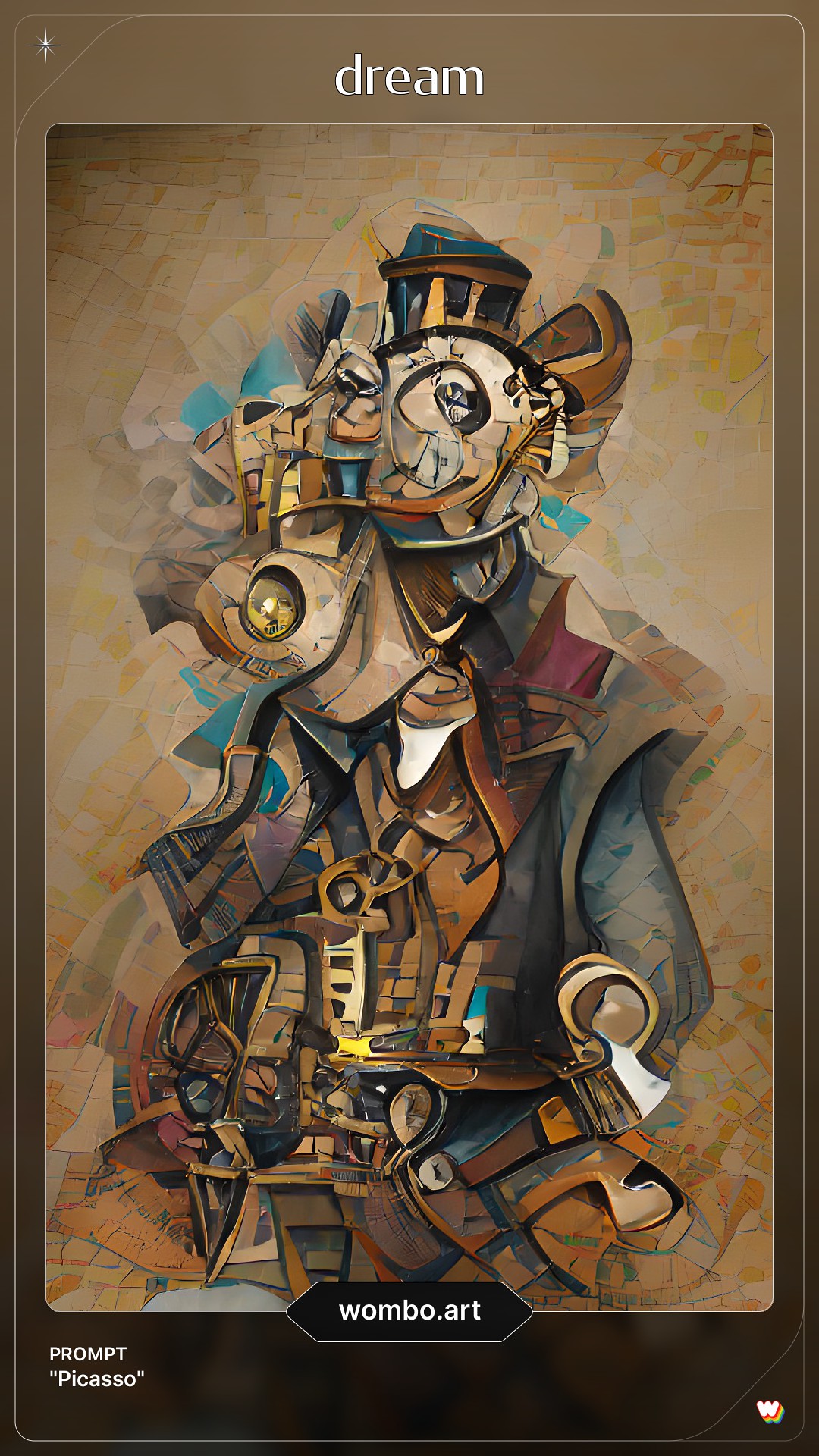This image showcases a striking piece of computer-generated artwork with a distinct Picasso-inspired style. The artwork features a primarily brown background, detailed with a complex array of vibrant colors—reds, blues, golds, yellows, and browns. At the top of the image, the word "Dream" is prominently displayed in white. 

The central figure, an abstract and deconstructed form reminiscent of a man, is composed of various shapes and elements that suggest both organic and mechanical features, giving it a robotic, almost metallic appearance. The figure includes a blend of forms, such as emanating sleeves, an implied necktie, and a vaguely defined head with the suggestion of a hat, all contributing to the dream-like composition.

At the bottom of the image, a cylindrical-triangle shape encloses the text "Wombo.art." In the bottom left corner, the words "Prompt: Picasso" are indicated in quotation marks, hinting at the AI-generated nature of the artwork. Additionally, a small red and white "W" logo is visible in the corner, further identifying the source of this digital creation.